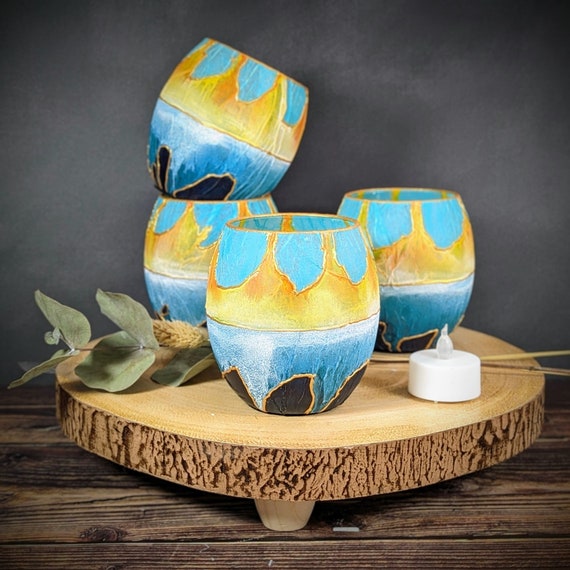This color photograph showcases a detailed and artistic arrangement of four ceramic cups displayed on a wooden platform. The platform itself features natural tree ring patterns on its circular top and bark-like textures along its sides, elevated by small wooden feet. This setup rests on an unfinished wooden table with a combination of light and dark brown hues. Each cup is predominantly decorated with blue and aqua blue tones, accented with yellow and black elements that resemble flower petals or leaves. Notably, one cup is nested within another, positioned at the left rear. Between the cups, there is a dried plant stalk with pale green leaves and a visible seed head, adding an organic touch to the composition. To the right of the cups, a cylindrical white object, possibly an electric candle, stands, featuring a translucent shape rising from its center. The entire arrangement is set against a dark gray wall, enhancing the visual contrast and focus on the details of the cups and the wooden textures.